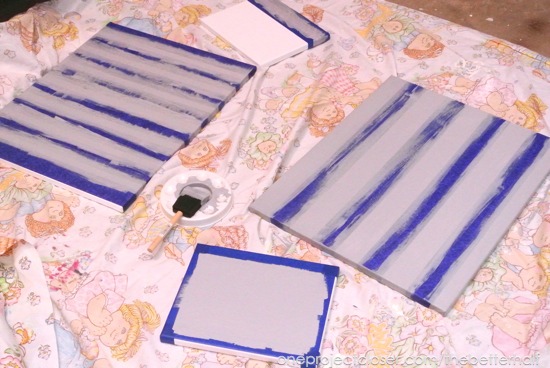The image showcases an arts and crafts project in progress, set atop an old sheet adorned with graphics of cartoon characters, including angels, flowers, and little girl dolls in colorful dresses of pink and blue. There are four painted boards arranged on the sheet—two larger and two smaller. The larger boards feature blue and gray stripes, while one of the smaller boards has a gray background bordered by blue paint. The other smaller board displays a white background with partial gray and blue stripes. Centrally placed among these boards is a small white lid or plate with a foam paintbrush resting on it, covered in gray paint. The brush handle is wooden and has a white label on it. Everything is set against a brown backdrop, contributing to the detailed scene.